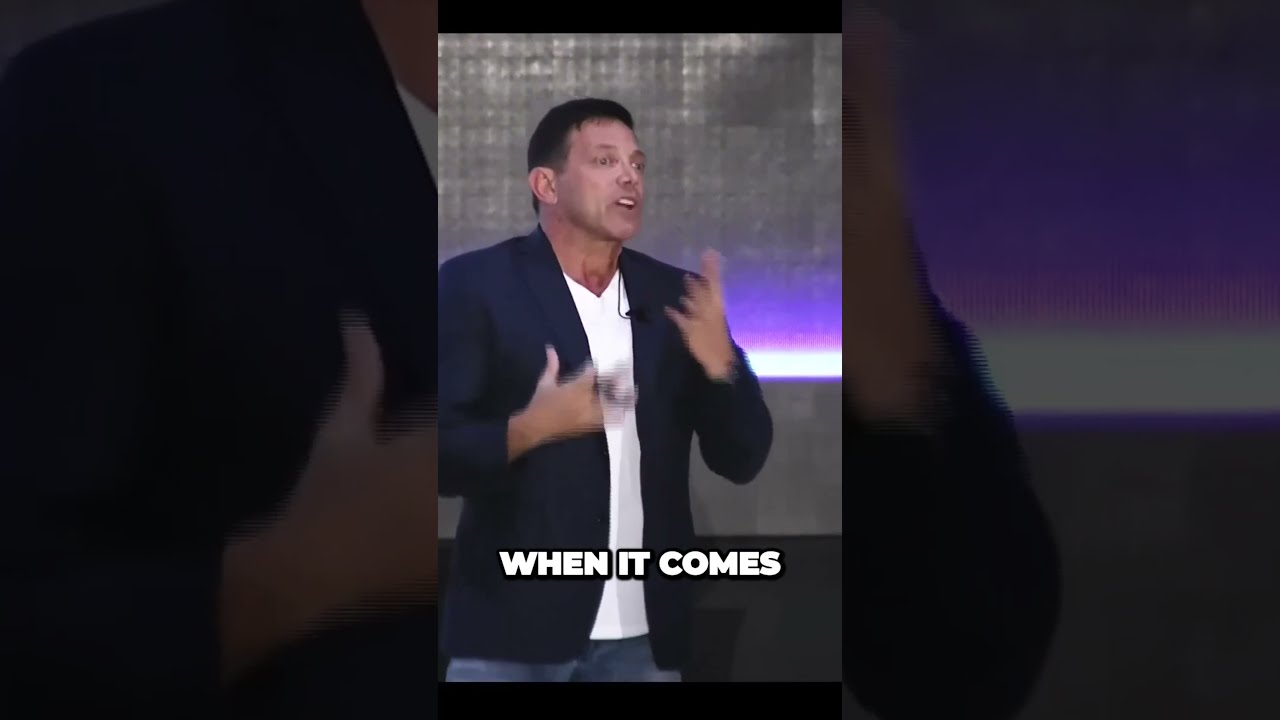The image is a horizontally rectangular shape divided into three sections: left, center, and right. The center section features a close-up of a man, appearing to be in motion. He has short, dark hair and olive skin and is wearing a white V-neck shirt under a blue or black suit jacket. His mouth is open as if he is speaking, and he appears to be gesturing with both hands in front of his chest. The blurred motion of his hands adds to the sense of dynamism. Superimposed across his waist in white letters are the words "when it comes." The background is a silvery gray with a purple bottom, with some parts appearing lit in white and purple light. The left and right sections are darker and enlarge parts of the man's body and hands, contributing to an impression of movement and focus.